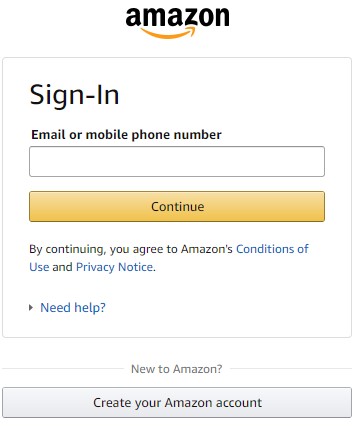The image showcases the familiar Amazon sign-in page, instantly recognizable to most people worldwide. Dominating the top of the page is the iconic Amazon logo, which sits prominently above the sign-in section. Directly below, the page prompts users to "Sign-In" and provides fields to enter either an email address or a mobile phone number. Positioned beneath this input area is a conspicuous "Continue" button.

Further down, links to the "Conditions of Use" and "Privacy Notice" are available for users who seek additional information on Amazon's policies. Adjacent to these links, a "Need Help?" button offers assistance to those experiencing difficulties with the sign-in process.

For newcomers, the page provides a clear call-to-action button labeled "Create your Amazon account," making it easy for new users to get started with Amazon. Despite the ubiquity of Amazon, the page remains prepared to welcome those rare individuals who are yet to join the platform.